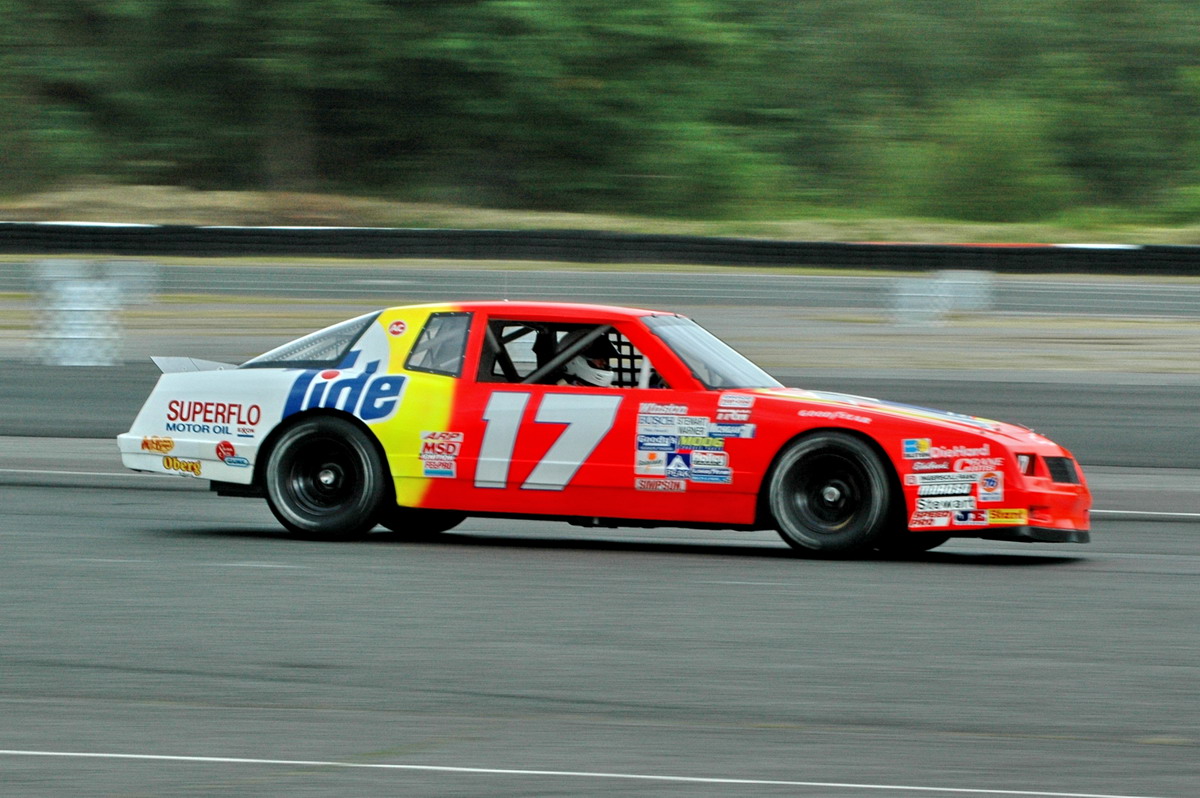This is a dynamic photograph capturing a high-speed stock car in motion on a racetrack. The image foreground features the gray racetrack, distinguishable by its white borders and stripes. In stark contrast, the background trees are rendered as green streaks, emphasizing the rapid movement of the vehicle. The stock car, predominantly orange from the doors to the front, features several sponsor logos, including prominent white "17" on the door. The rear third of the car transitions to yellow and white, displaying the Tide logo with its red dot above the 'i' and orange dot above the 'e'. Additional blurred sponsor logos like Bush, Moog, and Simpson are also present but less legible due to the car's speed. The overall high-quality photograph captures the essence of motion with the car appearing almost still against a backdrop of speed-induced blur.